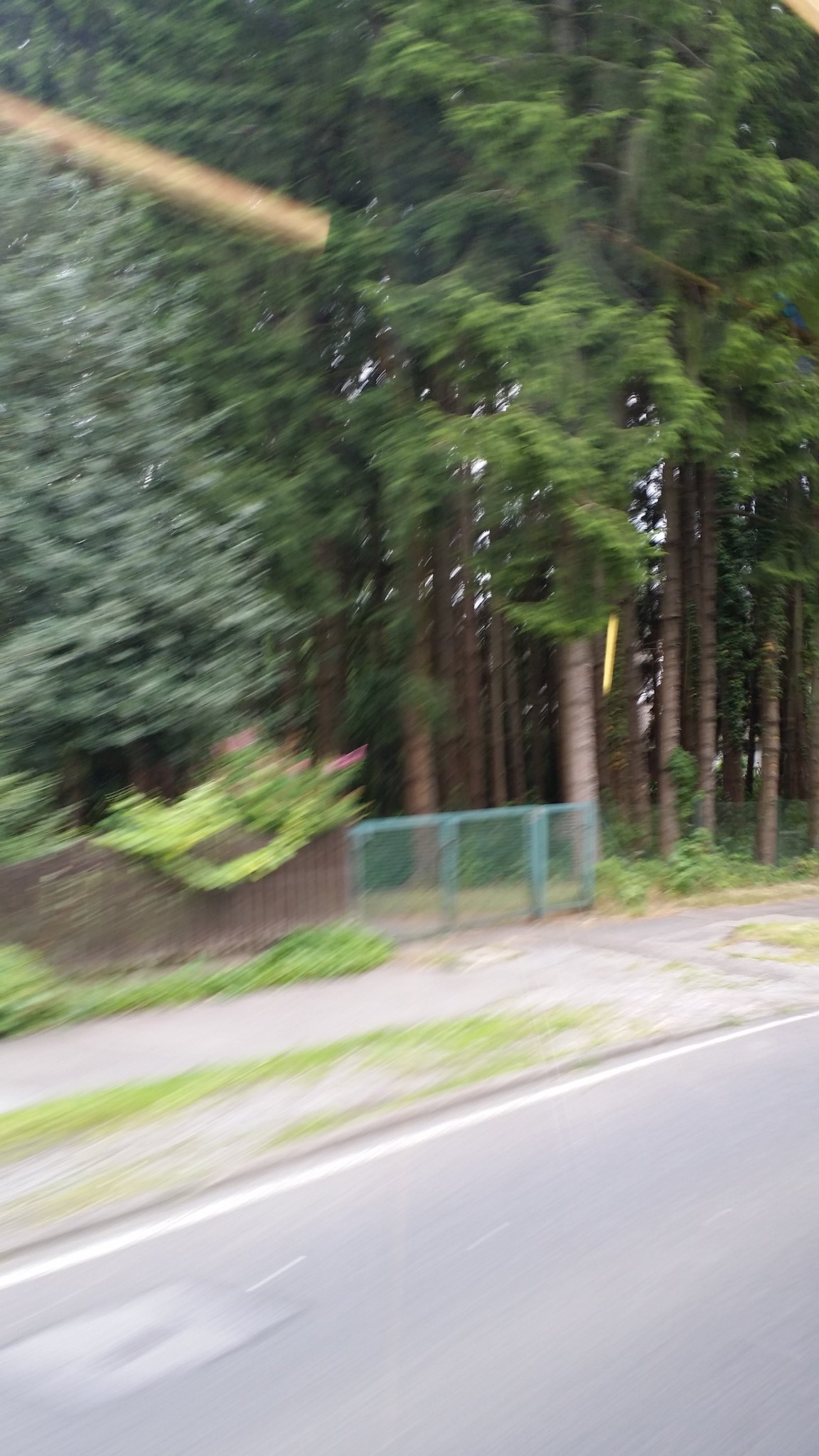The photograph depicts a somewhat blurry, outdoor scene captured through the glass of a vehicle, evidenced by an inexplicable light reflection in the upper left corner. The composition starts with a light gray asphalt road marked by a faint zero and bordered by a white line. Adjacent to the road lies a gravelly grassy strip followed by a gray concrete sidewalk. The sidewalk is intermittently dotted with patches of green grass and is flanked initially by low bushes against a brown wooden fence. This fence transitions into a green wire and metal gate, which is closed and leads to what appears to be a driveway. This driveway is backed by a dense wooded area populated with a variety of trees whose foliage ranges from bright mint green to deep hunter green. Some of these trees are adorned with pink flowers. Among the trees, vines are seen climbing parts of the brown fence. The tree trunks are predominantly light brown. Gaps in the foliage offer glimpses of a white sky, creating a complex interplay of natural elements in the middle and background of the image.